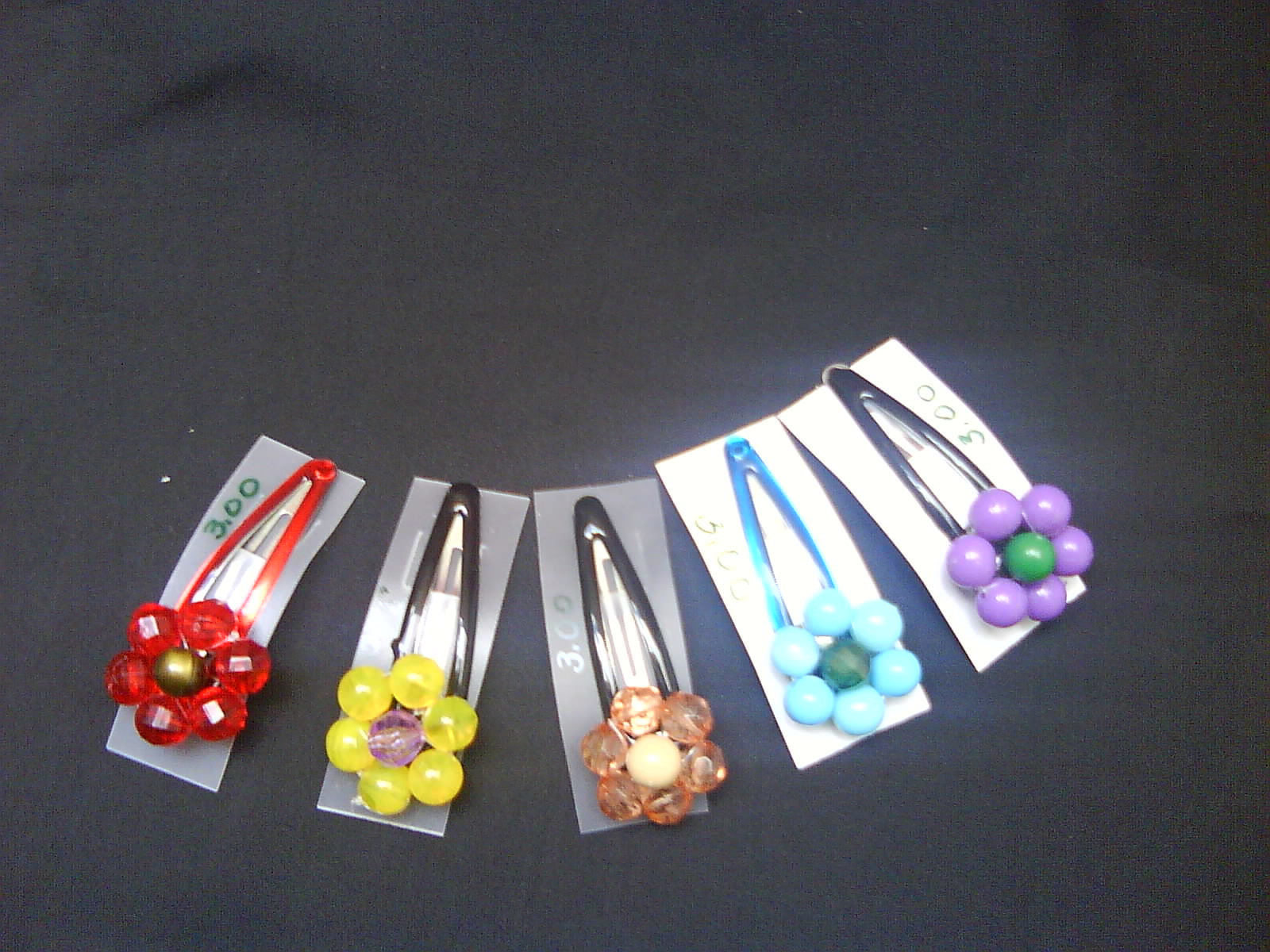The color photograph showcases a collection of five hair clips, or barrettes, arranged horizontally in a slightly upward-curving, fanned-out formation. Each clip features a beaded floral design with a central bead surrounded by six petals, and they are attached to rectangular backings that appear to be cardboard or plastic. 

From left to right, the first clip is bright red with a gold center, and it has additional white square decorations on the petals, anchored to a clip entirely red. The second clip has yellow bead petals with a light purple or lilac center, secured on a black clip. The third clip exhibits transparent orange petals with a yellow center, fixed on another black clip. The fourth is composed of pale blue petals with a central green bead, paired to a matching blue clip. Lastly, the fifth clip displays lilac petals with a green center on a black clip. 

These clips are set against a nearly black background, possibly a dark grey fabric with slight texture and indents, further accentuating the vibrant colors of the hair accessories. Small white flecks are noticeable to the left of the line of clips. Each clip's backing card partially reads "3.00," which likely indicates the price tag.